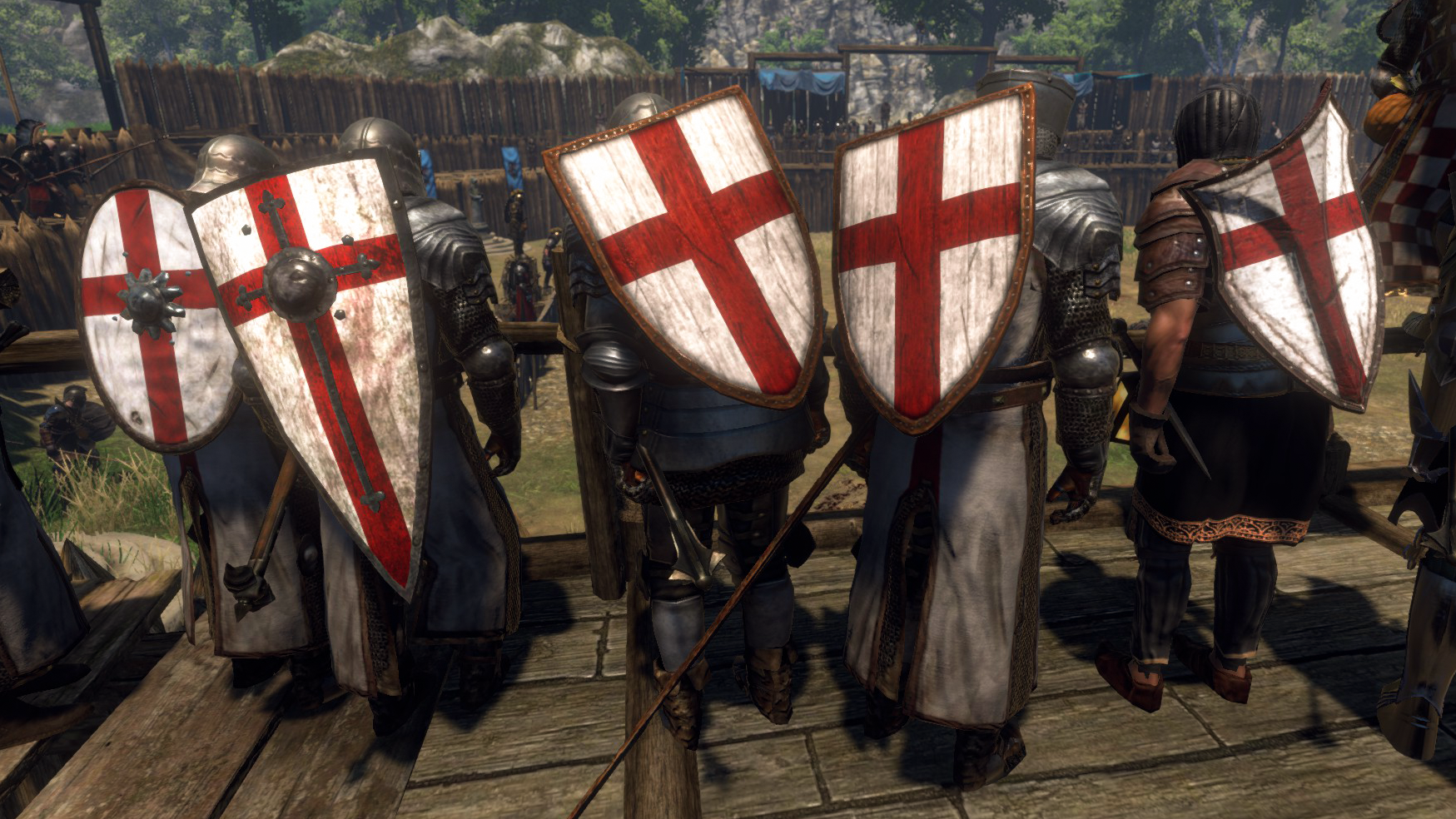The image depicts a group of five knights seen from the back, all wearing traditional armor with shields strapped to their backs. Each shield prominently features a red cross on a white background, with variations in shape and design: the knight on the far right has a round shield with a sun emblem, while the others bear V-shaped shields. They are wearing steel helmets, and one knight on the far right notably has a leather piece of armor, differing from the others' metal attire. The knights stand on a wooden platform, facing a fortified log wall that encloses a courtyard. The scene, possibly from a video game, shows the knights preparing to storm this fortress, their backs to the viewer, ready to engage the opposing force.